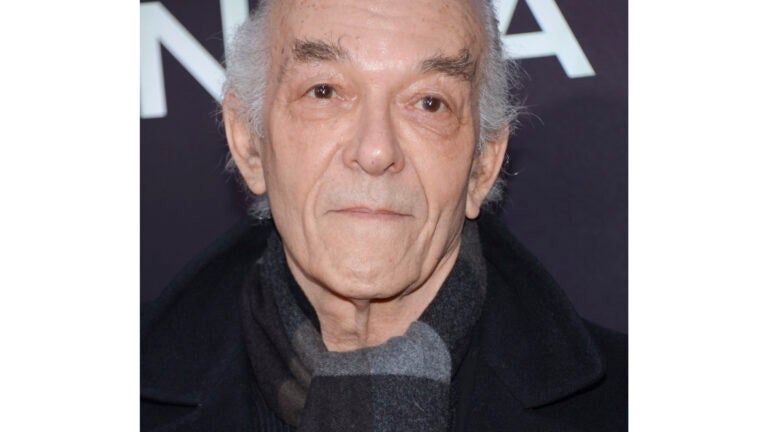The photograph captures a close-up of an elderly Caucasian man standing outdoors, likely at an event, evidenced by a dark blue banner with partial white lettering, including the letters "N" and "A", behind him. He is dressed warmly in a heavy black coat and a scarf that features a grey and dark grey square pattern. His stark white and grey hair, thinning on the top with more on the sides, contrasts with his dark brown, bushy eyebrows. His mouth is tightly pursed, revealing thin lips and a few wrinkles around them, giving him a worried or upset expression. He gazes just past the camera, not directly at it, and his large forehead is prominent against his minimal hairstyle. His scarf with blue and gray stripes and his jacket with a collar add to his dignified, albeit concerned, appearance.